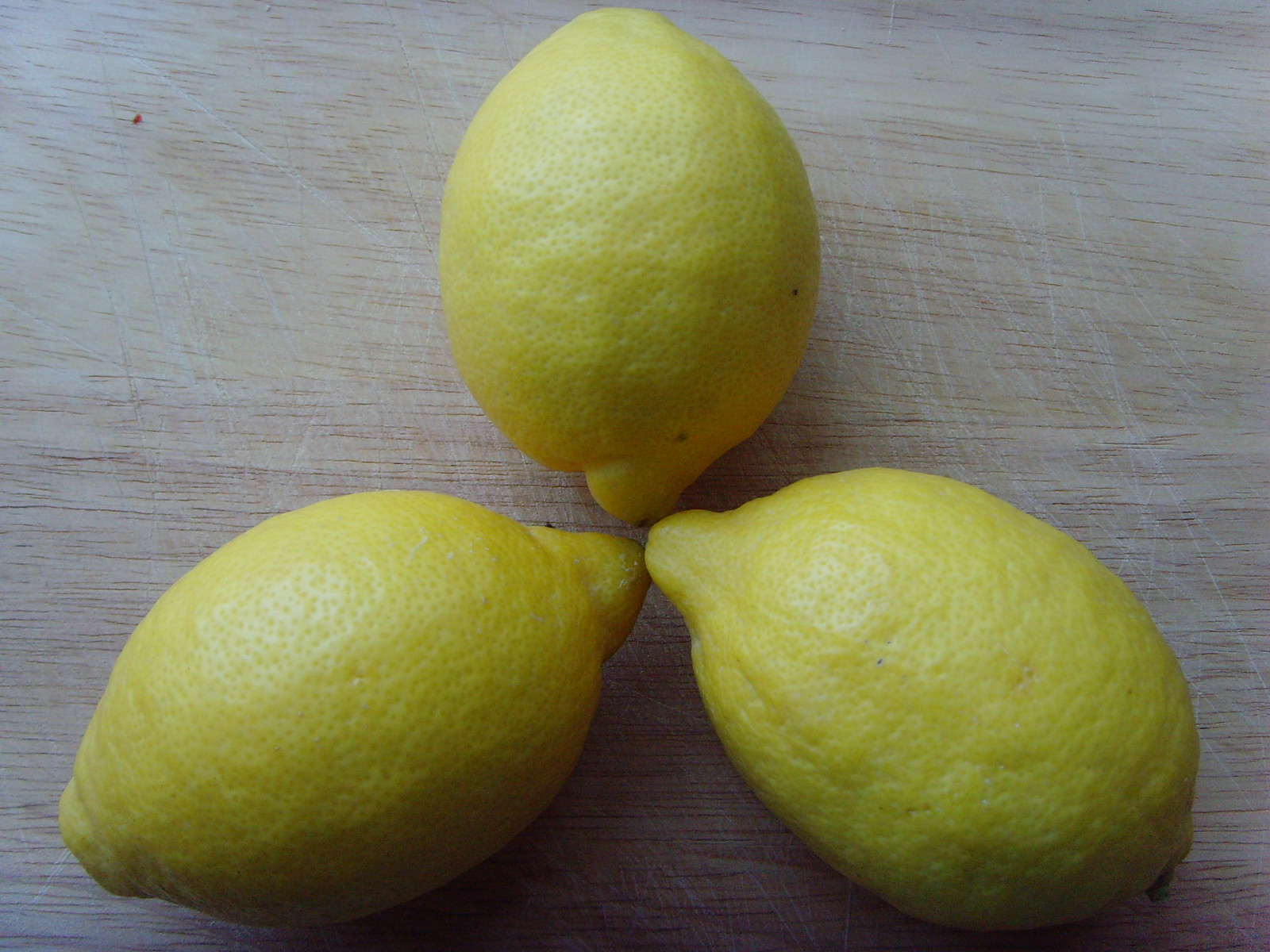The image is a color photograph taken from above, depicting three large, glossy lemons arranged on a light-colored wooden surface with visible grain running horizontally left to right. The lemons, positioned to form a roughly triangular shape resembling a trillium flower, are completely intact and untouched. The top lemon features a couple of small dark specks on its bright yellow rind, while the lemons at the sides exhibit slight shades of green and dark spots, along with sun glares highlighting their glossy textures. The wooden surface shows many scratches and cuts, imparting a well-used appearance. In the upper left-hand corner of the photo, a small speck of red, possibly a bit of food debris, is also visible.